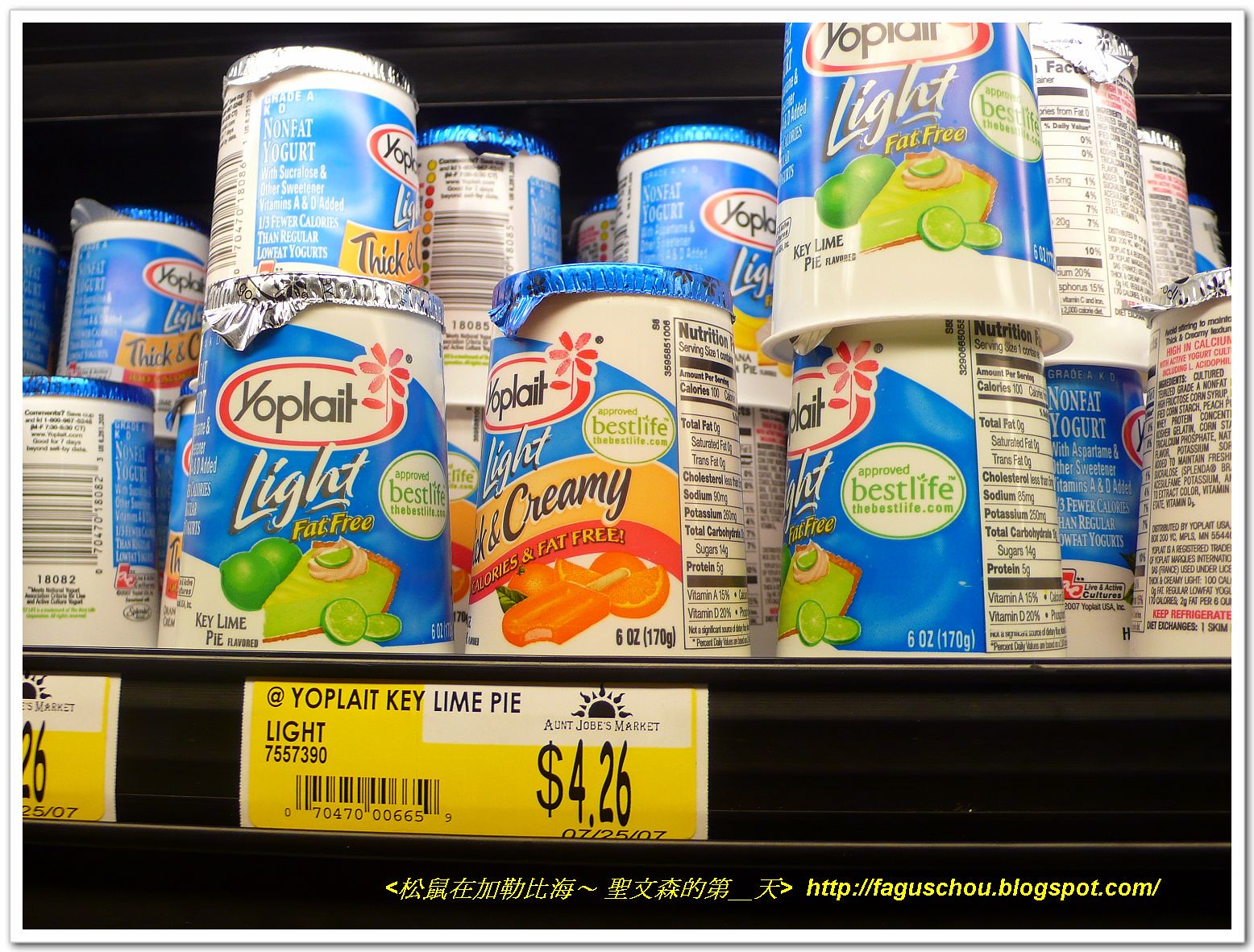This photograph captures a grocery store shelf displaying an assortment of Yoplait Lite yogurts. The shelf has a black front and features a yellow price tag listing "Yoplait Key Lime Pie Lite" at $4.26, with an oddly high figure of $75.57390 written before it. The yogurts are placed in white and blue containers with either silver or blue lids. Also visible is a light and creamy yogurt variant featuring an orange creamsicle design on the front. At the bottom of the image, there are some Japanese characters followed by the website URL: http://faguschou.blogspot.com/. Additionally, the shelf signage includes a Sunrise logo for "Aunt Jobe's Market." This detailed photograph, likely intended for a blog, showcases the available flavors and price details of the Yoplait Lite yogurt selection.